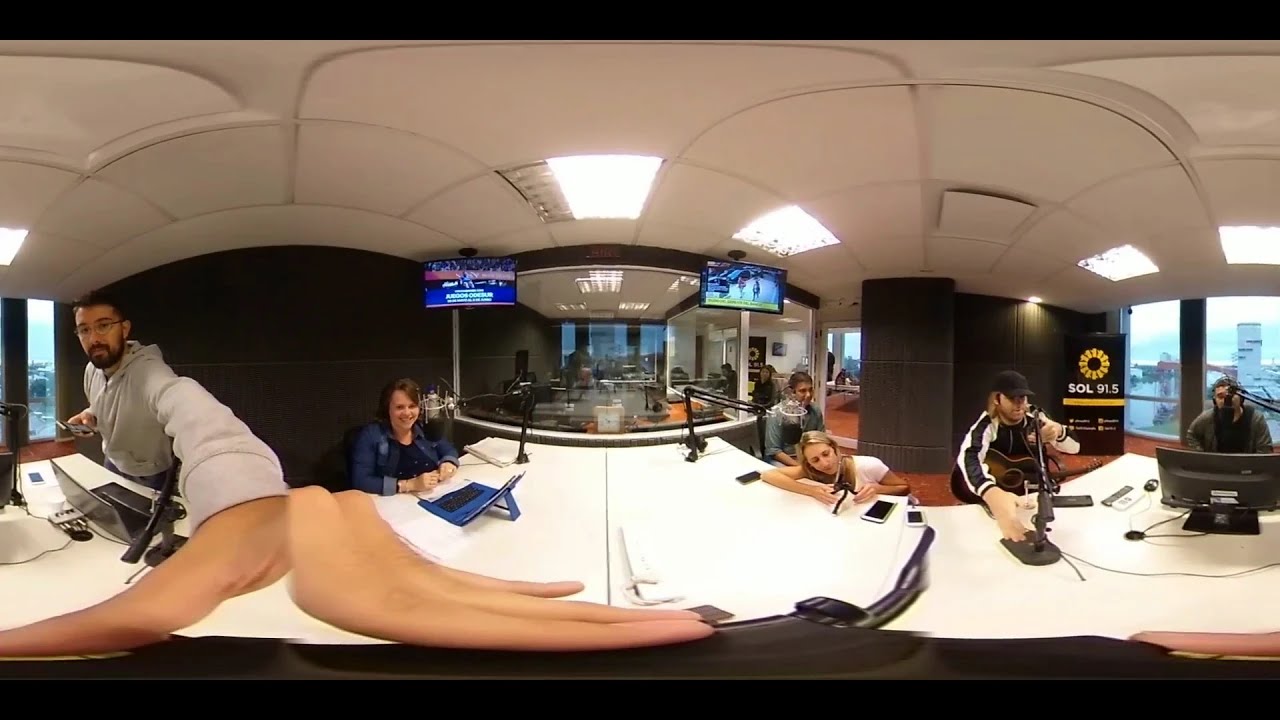The image is a highly distorted 360-degree shot of a professional radio station studio. At the forefront on the left, a man wearing a gray hoodie is leaning forward with his arm exaggeratedly stretched towards the camera, making his hand appear disproportionately large compared to his body. He has a black beard and glasses, holding a phone in his right hand and has a laptop in front of him. Seated next to him is a woman in a blue jacket, facing the camera with a laptop and a silver microphone on a black stand in front of her. 

Moving towards the right, the white table runs across the center with multiple black microphone stands. On the right side, there's another group of individuals: a man sitting and looking forward, a woman leaning on the table with phones in front of her, a man with an acoustic guitar adjusting the base of a microphone, and another man at the far right seated behind a computer monitor and microphone. 

In the mid-ground of the studio, there's a large glass window with two video screens hanging from the ceiling, which are turned on. Behind the glass, more office space is visible. Far to the right, through another window, skyscrapers are seen in the distance, indicating a city view outside. An orange circle with the text "Sol 91.5" is visible on a freestanding poster, reinforcing the professional branding of the station. 

Overall, the scene captures the hustle and bustle of the working environment of the radio station, filled with engineers, producers, and on-air talent amidst a multitude of technical equipment and professional ambiance.